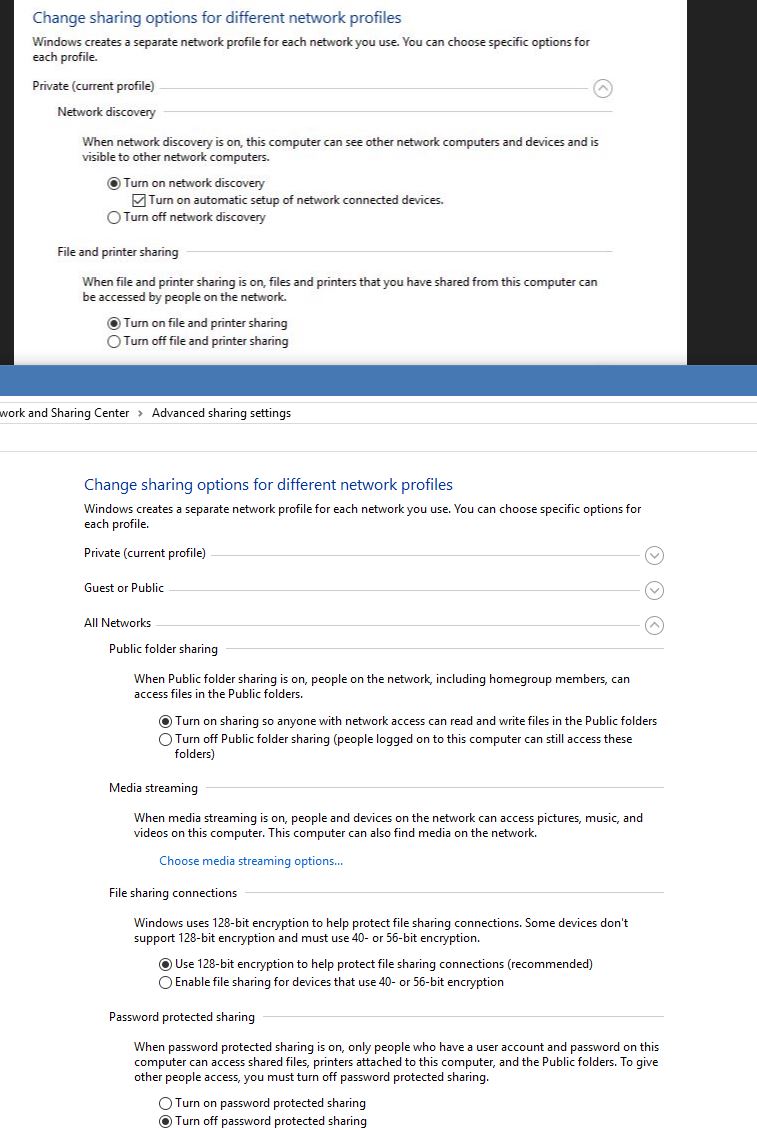This image captures a detailed view of a Windows network settings interface, specifically focusing on changing sharing options for different network profiles. At the top, the text explains that Windows creates a unique network profile for each network you connect to and allows you to customize settings for each profile.

In the first section, labeled 'Private (current profile)', there are options shown with bullet points. The first line is for 'Network discovery' and it is currently enabled, which means that this computer can see other devices on the network and is visible to those devices. The option 'Turn on network discovery' is checked off.

Following that, there's a section on 'File and printer sharing', with a description stating that when enabled, files and printers shared from this computer will be accessible to others on the network. The option 'Turn on file and printer sharing' is also selected.

This section is enclosed within a box featuring a thick black vertical line on the right, a thin black line on the left, and a blue bar running underneath it.

Below this, the interface repeats the header "Change sharing options for different network profiles" and provides further details categorized under 'Private', 'Guest or Public', and 'All Networks'. 

Each category presents additional options:
- **Public folder sharing**: Controls the sharing of public folders.
- **Media streaming**: Allows users to turn on media streaming and choose media streaming options. The text for this option is highlighted in blue.
- **File sharing connections**: It recommends using 128-bit encryption to secure file sharing connections.
- **Password-protected sharing**: Currently set to 'Turn off password-protected sharing', which means network users don’t need a password to access shared resources on this computer.

The comprehensive layout guides users through configuring their network sharing settings, ensuring both visibility and security preferences can be adjusted according to the selected network profile.